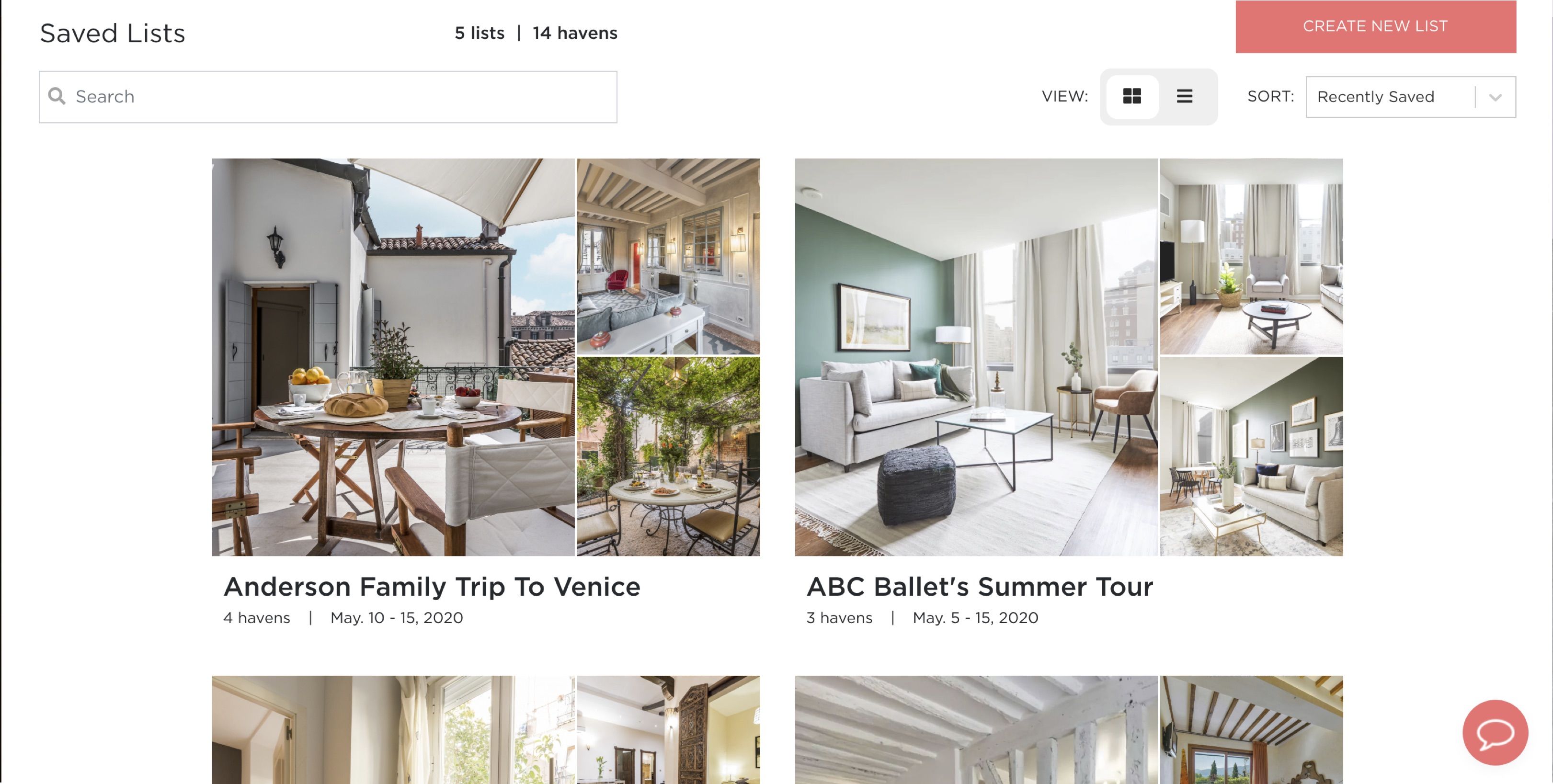The image showcases a user interface with various saved lists under a header that reads, "5 Lists, 14 Havens." Prominently featured is a red button labeled "Create a New List." There's also a search field available for users to refine their searches, accompanied by a "View" button and sorting options. The lists are currently sorted by "Recently Saved." A red message icon is visible on the interface, enabling users to contact someone from the website.

The first saved list is titled "Anderson Family Trip to Venice," which includes four havens scheduled for May 10th through the 15th, 2020. The accompanying image features a spacious outdoor eating area with a white house in the background, adorned with silver doors. The scene also highlights a pleasant living space and additional outdoor seating situated in a lush green area.

The second saved list is named "ABC’s Ballet Summer Tour," listing three havens for the period of May 5th through the 15th, 2020. The image for this list showcases various modern living spaces characterized by hardwood flooring and an array of white couches.